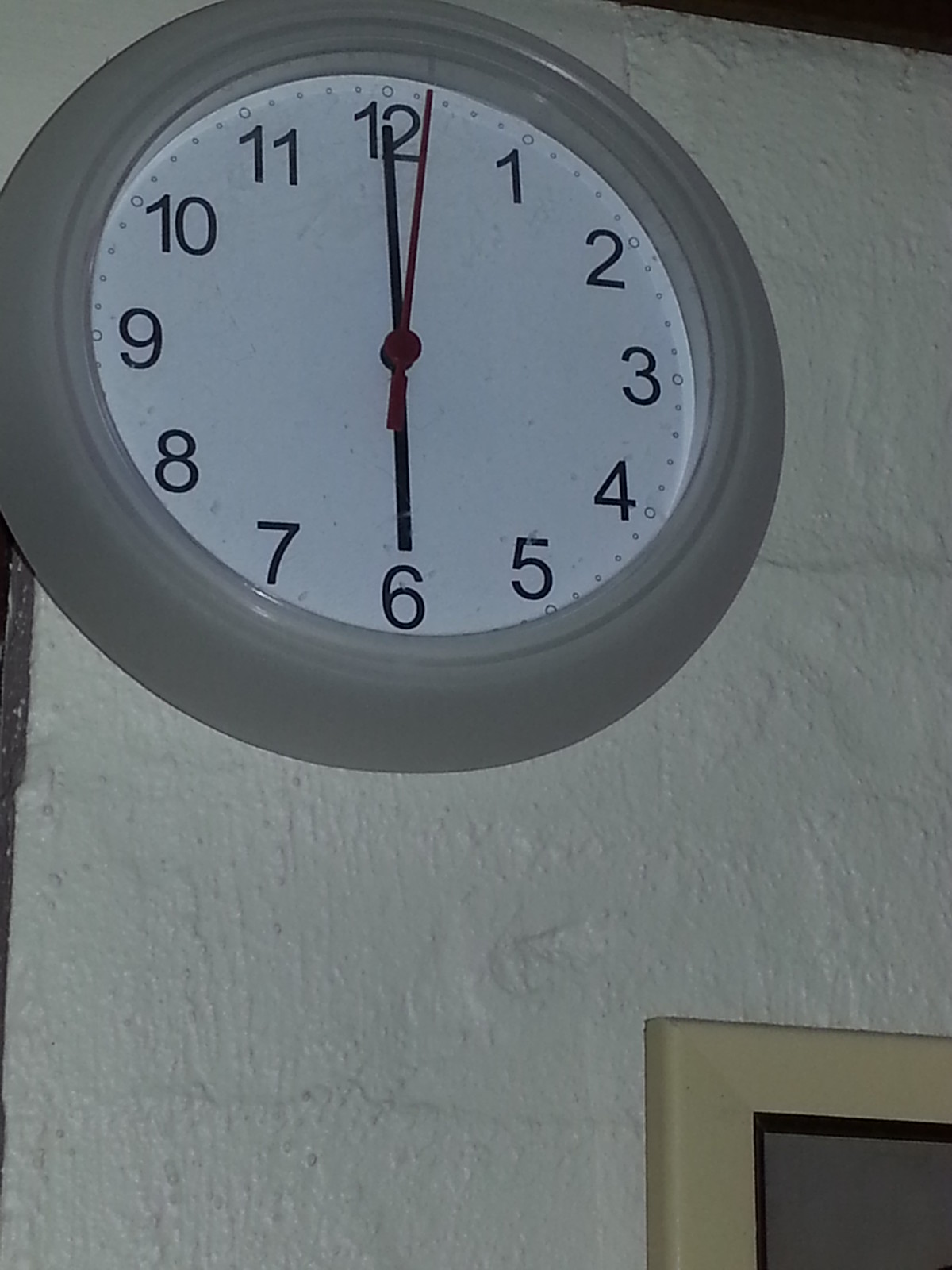The image portrays a wall clock affixed to a white cement block wall. The clock, which is round, features a thick, gray bezel. Its face is a clean white, adorned with black minute and hour hands, and a contrasting red second hand. The current time displayed on the clock is precisely six o'clock. The numerals on the clock face are in traditional Arabic numerals, providing clear and easy readability. On the bottom right edge of the photo, there is a doorway or door partially in view. This doorway includes a square frame and what appears to be another 90-degree frame inside it, with a brown square element centrally located, likely indicating a wooden door or a similar feature.